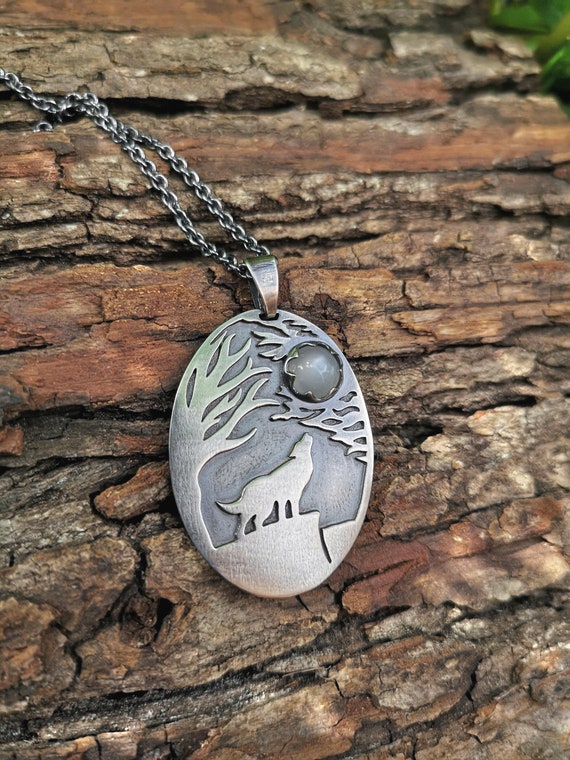This image features an intricately designed necklace with a silver chain. The focal point is an oval-shaped pendant made of dark grayish metal, resembling steel. The pendant features a detailed carving of a wolf howling at the moon, standing atop a cliff. Surrounding the wolf are branches and trees, evoking a woodsy scene. The moon is depicted with a round gemstone, possibly a pearl, adding a luminous touch to the piece. The necklace is photographed against a textured dark brown tree bark, enhancing the natural, earthy theme of the pendant's design.